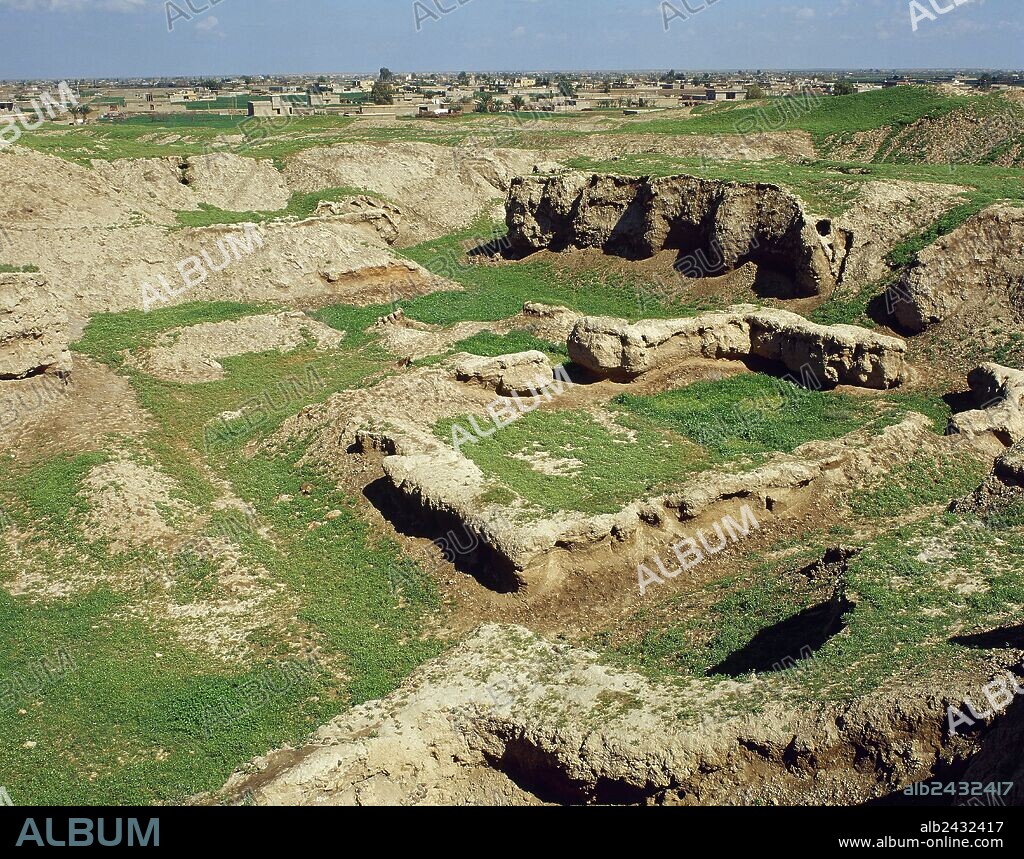The photograph, captured from an elevated vantage point on a sunny day, depicts a landscape featuring ancient ruins interspersed with patches of dense green bushes and light dirt areas. Some of the wider dirt sections rise up, resembling stone formations with a gray tint. The distant background shows a flat horizon with clear, light blue skies and scattered buildings, possibly villages or neighborhoods. Dominating the image are multiple watermarks of the word "album," in both white and lighter gray, suggesting the image is owned by a company named Album. At the bottom of the photo, a black stripe includes the word "album" on the left and "ALB 243-2417 www.album-online.com" on the right.